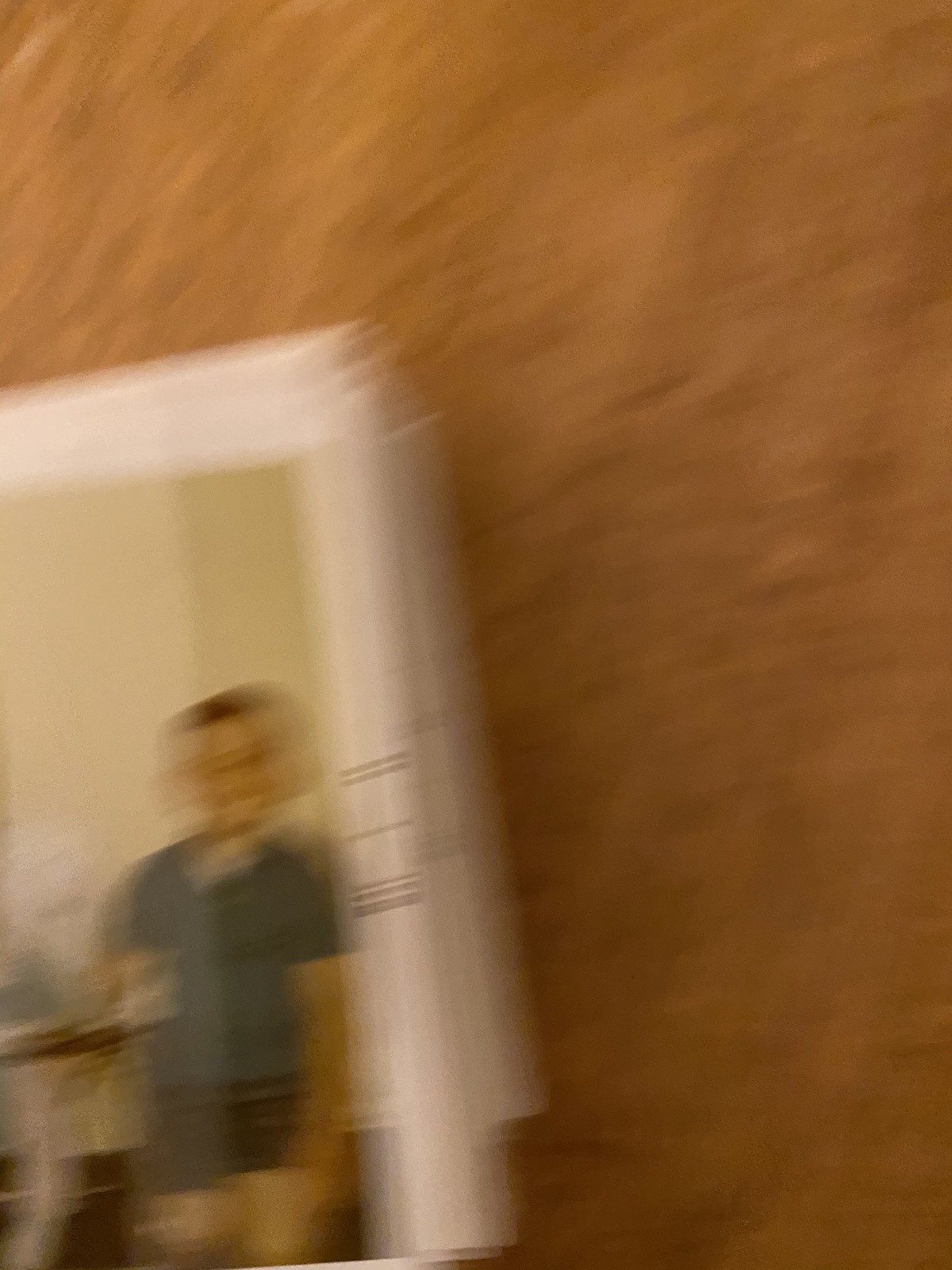The image depicts an extremely blurry snapshot of what appears to be a stack of old photographs, possibly Polaroids, lying on a textured surface that might be a piece of fabric, carpet, or a tabletop with a tannish-brown color. The top photo in the stack shows a young boy with short brown hair, wearing a bluish-gray or dark blue-green short-sleeved shirt and black shorts. The boy seems to be leaning on the edge of a table. Due to the blurriness, details are difficult to discern, but the white border of the photo is visible along with some faint black numbers, possibly a date stamp commonly found on older prints.